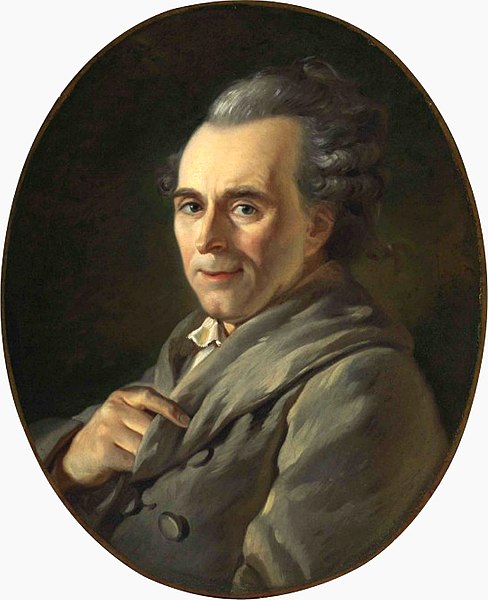This is a detailed color portrait painting titled "Portrait of Michel-Jean Sedain," created by Jacques-Louis David in 1772. The artwork displays an elderly Caucasian man in his late 60s or 70s, depicted from mid-chest up, within a white rectangular frame that encapsulates a dark oval background of almost blackish brown and green hues. The man is seated with his body angled to the left, his head turned to the left but looking directly at the viewer with gray-blue eyes, a slight smile, and a dignified expression. His gray hair, brushed back and curling on the sides, recedes into a widow’s peak. He has a lined face, a straight narrow nose, a cleft chin with a bit of five o'clock shadow, a slightly longer space between his nose and thin upper lip, and a healthy reddish-pink lower lip. He wears a heavy olive green overcoat with a hint of a white ascot or collar peeking out, and his right hand is positioned with three fingers inside the coat, the index finger resting on the lapel. The style of the painting is characterized by oil painting realism in a vintage aesthetic.